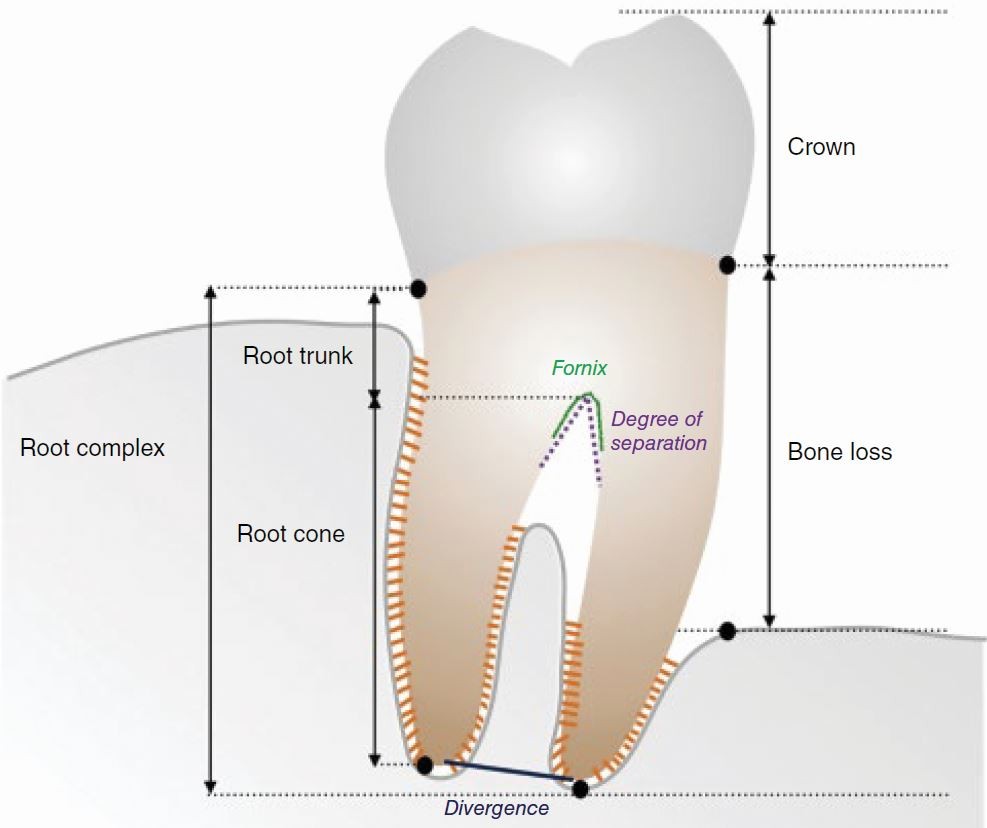This detailed diagram of a tooth, possibly from a dental textbook, showcases a side view of a tooth embedded in the gum. The diagram delineates several key parts of the tooth and the surrounding structures. The top part of the tooth, labeled "crown," is depicted in a light gray color, while the roots, referred to as "root trunk," "root cone," and "root complex," are colored a yellowish beige. The gum surrounding the tooth is shown in a solid light gray.

The image also highlights "bone loss" near the bottom part of the tooth. Detailed annotations call out various elements, including "divergence," which measures the distance between the two prongs of the roots, and "degree of separation," indicating the space where the roots bifurcate, labeled at the fornix with green text. The fornix is marked with a green arc beneath it and a blue upside-down V in dotted lines pointing upwards.

In the background, there is a gradient of light blue fading into white at the lower parts of the image. The gum line is particularly described with a complex, bluish-gray line that curves and winds across the diagram, reinforcing the separation between the gum and the tooth. The diagram uses black dots and skinny black arrows to highlight specific parts of the tooth, with the arrows indicating directions from the top to the bottom.

The crown at the top of the tooth is represented with lobes and valleys, shaded blue with white in the center. The roots, taking up about two-thirds of the tooth, are depicted with burnt orange lines radiating around them, resembling small ladder rungs. These elements collectively provide a comprehensive visual guide to the structure and condition of the tooth within the gum.